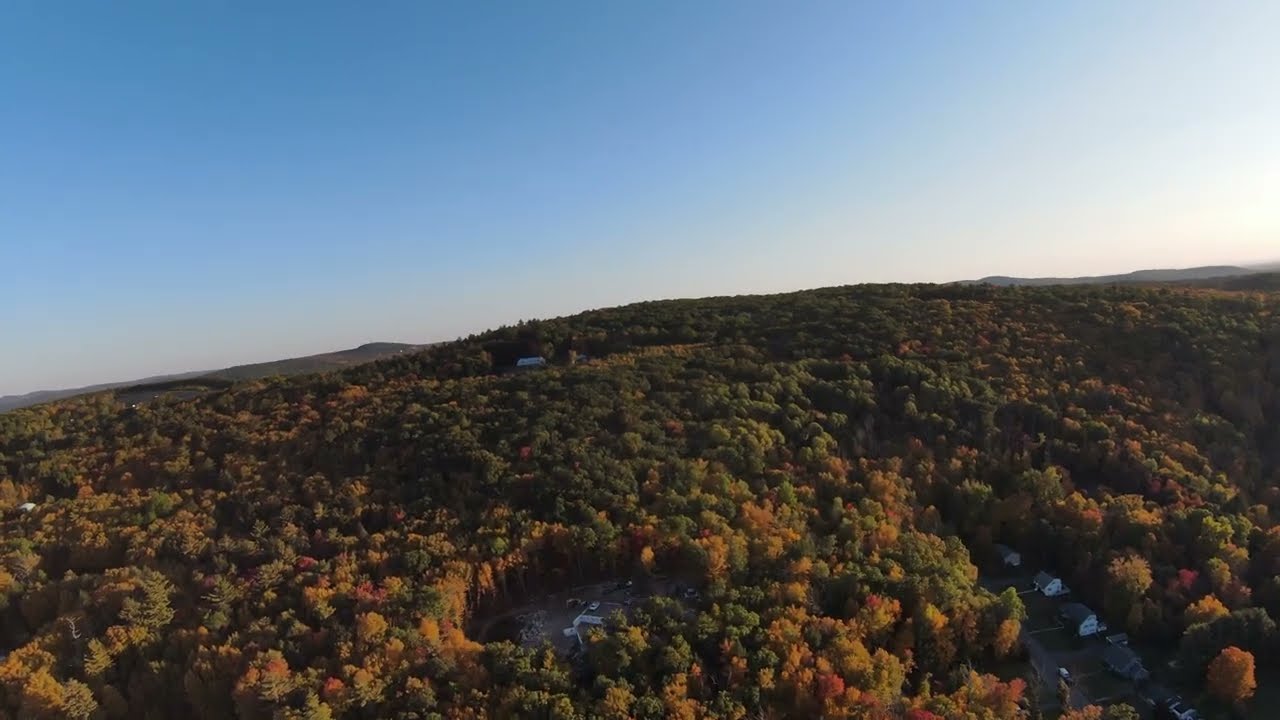This detailed aerial shot, possibly taken from a drone, captures a picturesque hillside and forest during the fall season. The richly colored foliage dominates the landscape, showcasing a stunning array of yellows, oranges, reds, and deep greens from evergreens that stand resilient against the autumn change. Nestled atop the hill, a solitary house is bordered by dense forest. As the hillside descends, a large clearing midway reveals another white house. Further down, another extensive forest spans the area until two white, identically designed houses appear in a second clearing. The lower right of the image features a well-maintained neighborhood with similar style homes arranged in a cookie-cutter pattern. The background is adorned by an expansive mountain range extending across the entire photo, under a crisp, cloudless blue sky. The highlight of the image is undeniably the vibrant fall foliage, painting the scene with natural autumnal beauty.